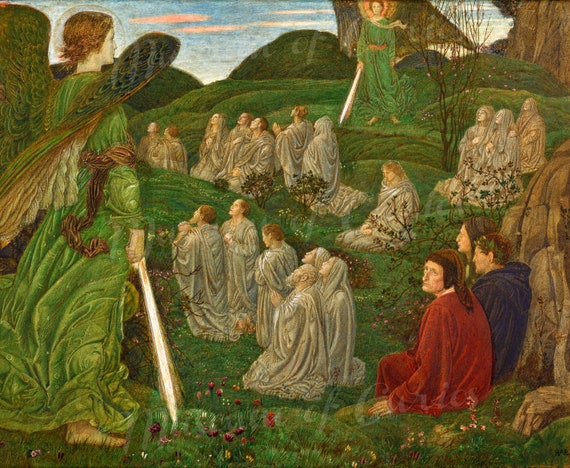The digital drawing, created in a style reminiscent of medieval art, depicts a serene landscape characterized by a blue sky with a few clouds and green hills in the background. The foreground features a grassy field with mounds, and on the right side, a notable rock. Standing nearby are three figures: one in a red cloak and hat gazing to the left, another in a blue cloak with a crown of flowers, and the third partially obscured, showing just their face near some bushes. Dominating the left side of the image is an angel dressed in a green robe with a sash, wielding a downward-pointing sword. This angel, with reddish hair and wings, is mirrored by another similar angel in the distance, also holding a sword. Central to the composition are two lines of men and women in white robes, all looking upwards in prayer, suggesting a spiritual gathering. The overall scene gives an impression of divine presence on Earth, blending piety with a touch of the supernatural.